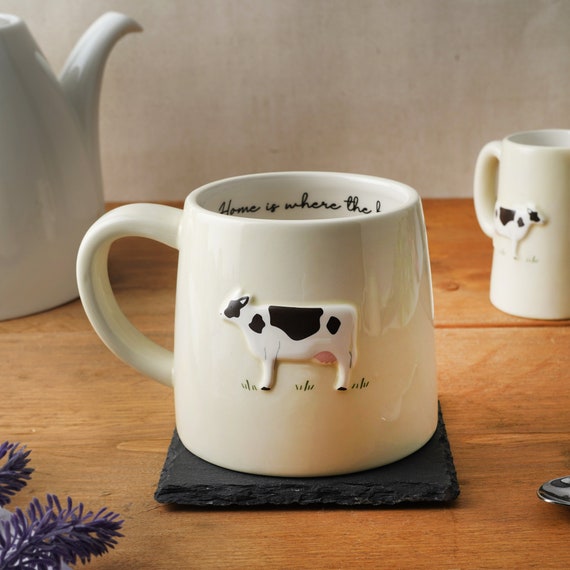The image depicts a detailed and carefully composed scene, likely intended for a food magazine or advertisement. Central to the composition is a short, wide-based porcelain mug adorned with a raised black-and-white cow motif, complete with detailed features such as a black spot on its back and simulated grassy lines beneath its feet. Inside the upper rim of the mug, the cursive inscription "Home is where the" is visible. The mug is placed on a black stone coaster, all set against a rustic wooden table. Surrounding the central mug are slightly out-of-focus objects: to its left, there's a hint of a white teapot, while to its right, a similarly designed mug or possibly a creamer cup can be seen. A purple plant's foliage enters the frame from the bottom left corner, adding a touch of color, and the tip of a spoon peeks in from the bottom right corner. The soft lighting accentuates the centerpiece, giving the image a warm, inviting feel.